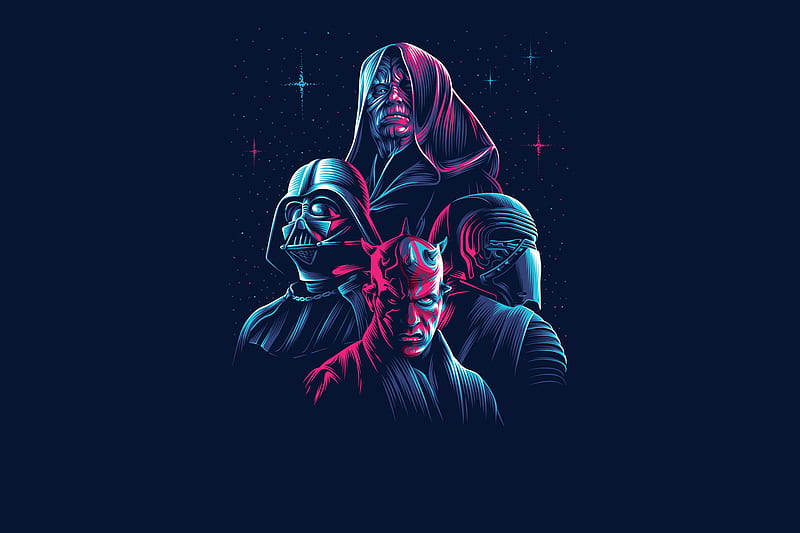This detailed image features four iconic characters from the Star Wars franchise, arranged in a unique, stacked profile view from shoulders upwards. The background is a deep, dark blue adorned with multiple four-pointed starbursts in shades of blue and purple. The color palette of the characters themselves primarily uses red and blue.

At the bottom is Darth Maul, easily recognizable by his black robes, red face markings, and horns protruding from his bald head. To his right stands Kylo Ren, wearing his characteristic black helmet with a visor and black robes. On the left side of the middle row is the imposing figure of Darth Vader, clad in black armor, a large black helmet, and a rebreather mask. At the top, a Sith Lord wearing a hooded black robe completes the scene. The characters exude a sense of menace and mystery, enhanced by the vivid magenta highlights and the starry backdrop that evoke a sense of cosmic grandeur.